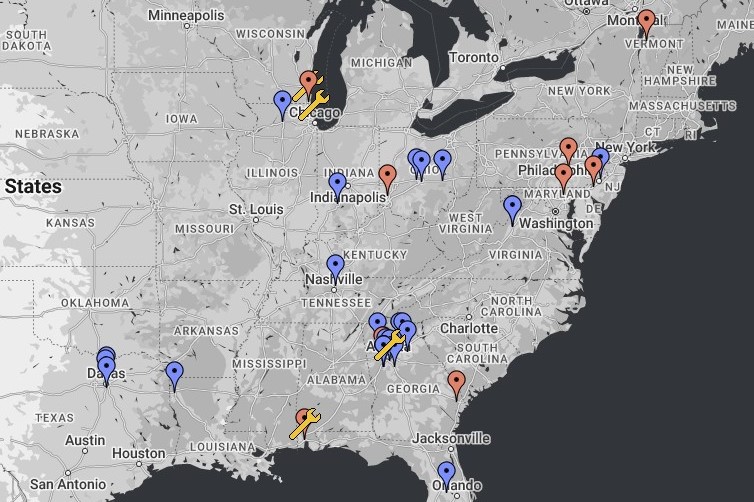This grayscale map of the United States is densely populated with different colored location markers, likely from a business website displaying its various office or service locations. The map primarily focuses on the Eastern and Central regions of the U.S., extending from the Northern States, such as Wisconsin, Michigan, and New York, to the Southern tip of Florida, and from the Central States, including Texas, Oklahoma, Kansas, and Nebraska, across to the Eastern Seaboard. A small portion of Southern Canada is also visible at the top.

The map features three distinct icons: a blue pin, a red pin, and a yellow wrench. These markers are dispersed across multiple key areas. For instance, numerous pins are concentrated around Atlanta, Georgia, the Northeast covering cities like Philadelphia and New York, and the Midwest around Indianapolis and Ohio. Other clusters are seen in the Southeast near Orlando, Southern Georgia, and Alabama, as well as in the Southwest, particularly around Dallas, Texas.

The states are illustrated in varying shades of light gray, while bodies of water such as the Atlantic Ocean, the Gulf of Mexico, and the Great Lakes are depicted in dark gray, enhancing the contrast and readability of the markers. This visually informative map provides a clear indication of the company's widespread presence across significant urban centers and regions in the United States.